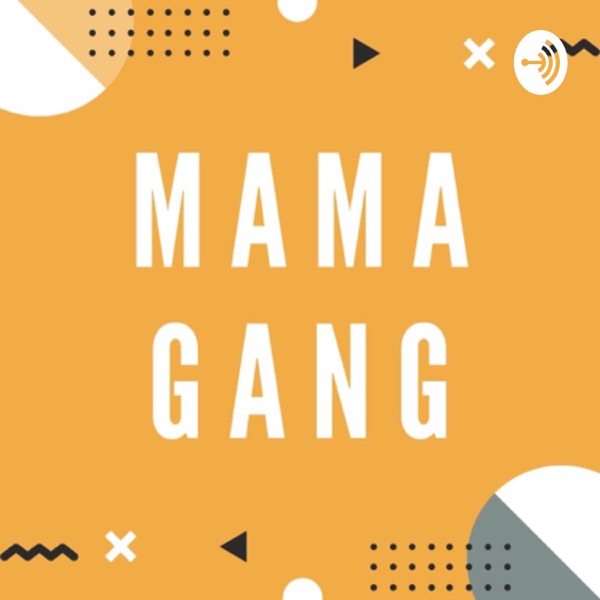The image features a predominantly orange square logo with detailed and intricate elements positioned methodically across its composition. The center prominently displays the text "MAMA GANG" in large, white, capital letters that span two lines. The logo incorporates several consistent shapes and symbols in black, white, and gray, which stand out against the vibrant orange background. 

In the upper left corner, there is a distinctive circle divided into two halves—one white and the other tan—accompanied by three rows of black dots. Adjacent to this circle, moving rightward, lies a black play triangle and a white 'X' symbol. The upper right corner also features an additional logo.

The lower portion of the image mirrors the upper arrangement. Starting from the lower left, there are black wavy lines followed by another white 'X' and a black play triangle, this time oriented in the opposite direction. Further right sits another half-circle—gray and white—also accompanied by three rows of black dots. The entire backdrop, though predominantly orange, includes noticeable notches at specific intervals, adding an extra layer of visual interest.